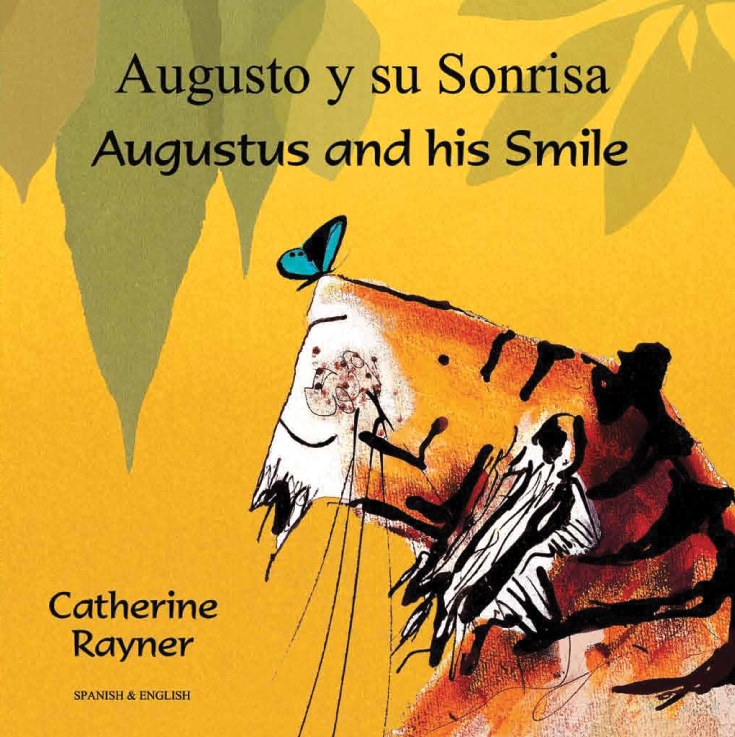The image depicts the cover of a bilingual book titled "Augusto y su sonrisa," or "Augustus and his smile," by Katherine Rayner. The cover features a childlike, distorted drawing of a lion, marked with the typical yellow fur and black lines but appearing very scribbled and disjointed—making it difficult to distinguish specific features like the eyes, nose, and mouth. A blue and black butterfly is perched on what appears to be the lion's nose, adding to the whimsical feel of the illustration. Surrounding the central image are green and orange leaves, set against a bright mango yellow background. The overall appearance is informal and playful, echoing the style of children's drawings.